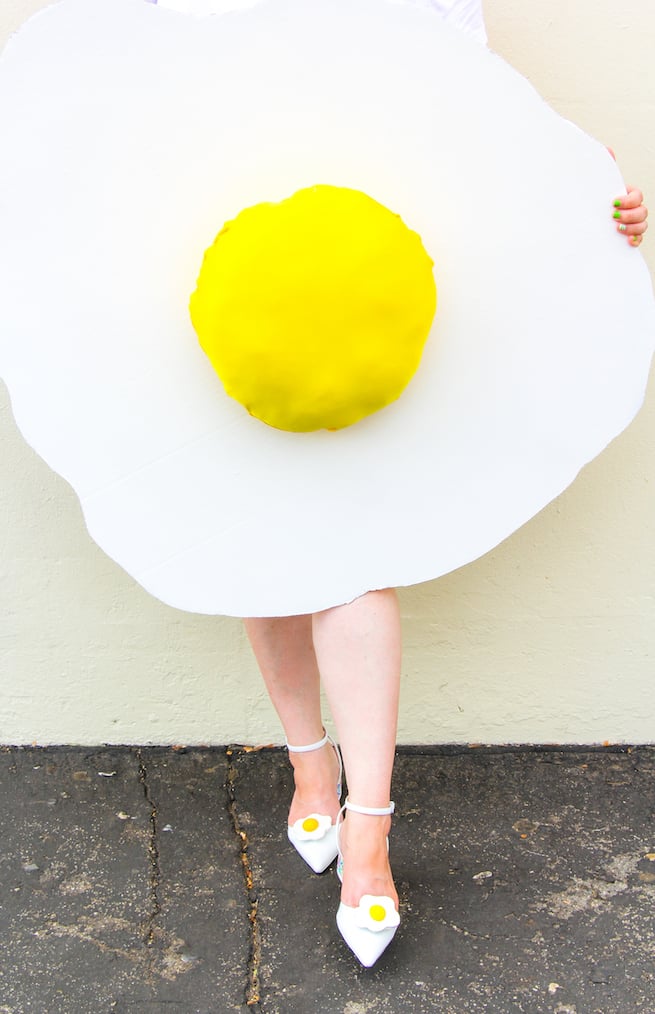In this outdoor image, a woman stands on a black and gray, crack-riddled asphalt surface, in front of a white wall. Her feet are adorned with white shoes, each featuring a design of a sunny-side up egg. Only her legs and left hand are visible, as her upper body is completely obscured by a large cut-out whiteboard, shaped like a sunny-side up egg, with a round yellow center. Her left hand, with green-painted nails, is seen gripping the top right corner of the whiteboard. The scene highlights the dirt and wear on the ground, adding a gritty texture to the overall composition.